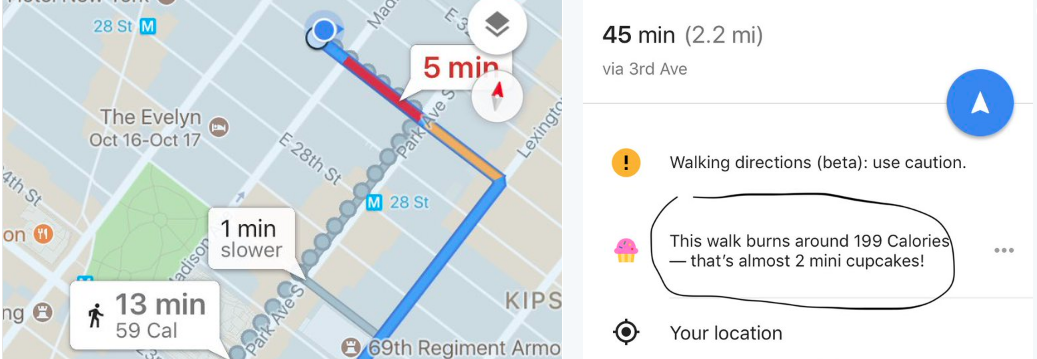This detailed caption describes an image captured from a navigation application, likely Google Maps, portraying both a map and various user interface elements:

---

The image displays a map interface, segmented into two distinct sections. The left portion features the map itself, primarily shaded in a light bluish hue. Prominent on this map are several wider, white-colored roads running diagonally from the top towards the left, intersected by thinner roads that extend from the right upwards to the left. A small green section, indicative of a park, is situated about two inches from the bottom left corner, partially overlaid by various icons and text.

Near the bottom of the map overlay, there's a dialogue bubble displaying "13 minutes, 59 Cal" accompanied by a walking icon, with a note stating "1 min slower" to the right. From the top center of the map descends a blue route line which transitions into a red line after about a quarter-inch, followed by a yellow line stretching approximately an inch and a half. This route then angles off towards the bottom left of the page, converting back to a blue line. Above the red segment, a pop-up icon reads "5 minutes" marked in red. Adjacent to this, two small circles are evident: a white one with a black square and another white circle featuring a red arrow pointing upwards, inscribed with "69 Regiment ARMO". Street names in black text are scattered across the map.

On the right side of the image, the background shifts to pure white. Adorning the top-left of this section, the text states "45 min" followed by "2.2 miles" in parentheses, and directly below, the route description via "3rd Avenue". Dominating this area is a large blue circle with a white upward arrow, below which lies a yellow circle marked with a black exclamation point and labeled "walking directions, beta, use caution". Further down, a whimsical cupcake icon, pink on top and yellow at the bottom, is encircled with a pin that declares "This walk burns around 199 calories". Below this, a playful remark asserts "that's almost too many cupcakes". Finally, at the bottom, a location icon accompanies the text "your location" in black.

---